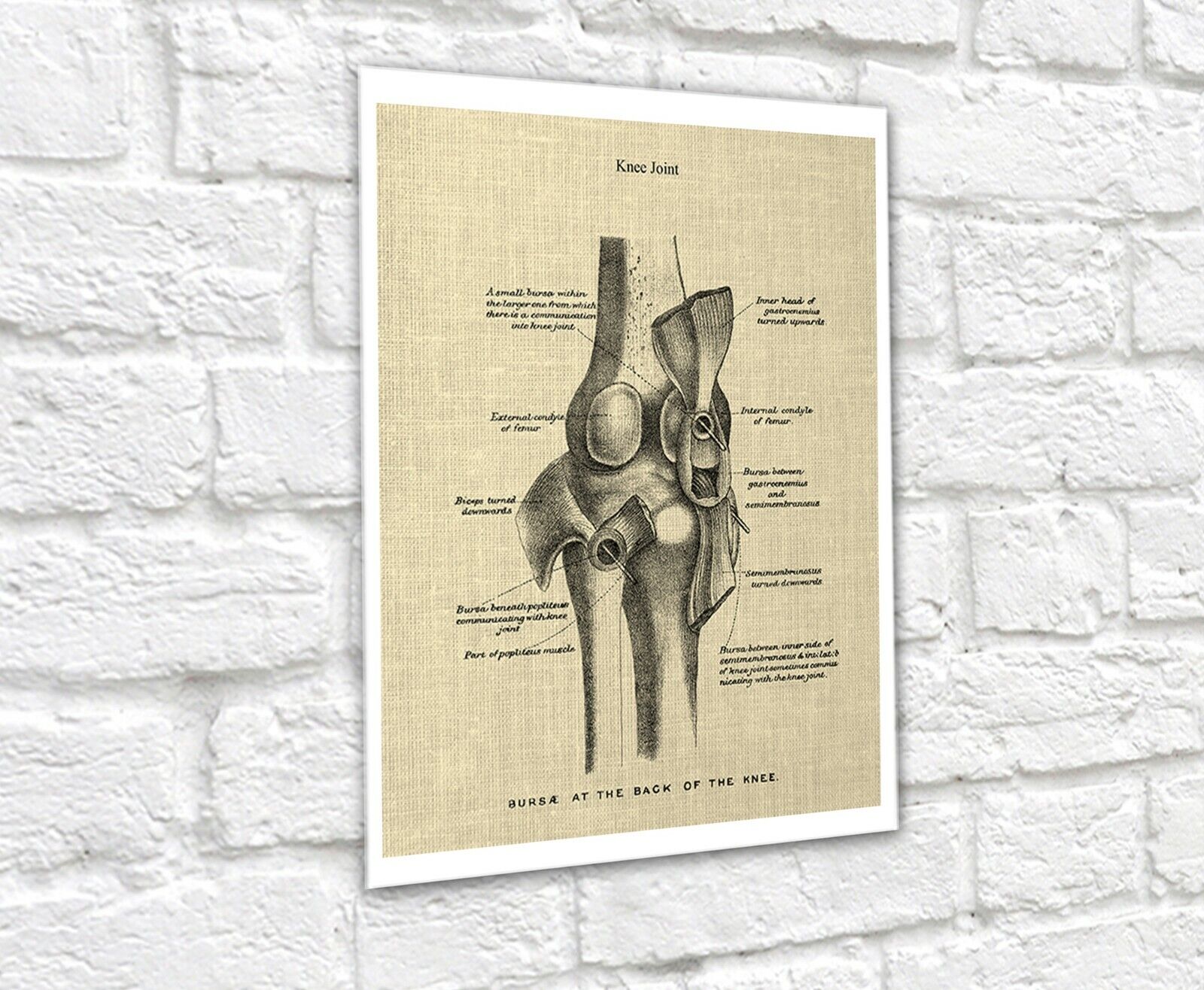This image showcases a detailed, black-and-white medical illustration of a knee joint, prominently labeled "knee joint" at the top and "Bursa" at the bottom. The illustration appears to be a 3D cross-sectional view of the knee, with various parts labeled, including the internal condyle of the femur, external condyle of the femur, and internal head, though the text is somewhat blurry. This drawing is rendered on what appears to be a beige, linen-textured rectangular piece of paper that gives off an aged, vintage look. The illustration is framed by a white border and casts a slight shadow, adding to its superimposed appearance on a white-painted brick wall, which enhances the sense of it being photoshopped onto the photograph rather than physically present.